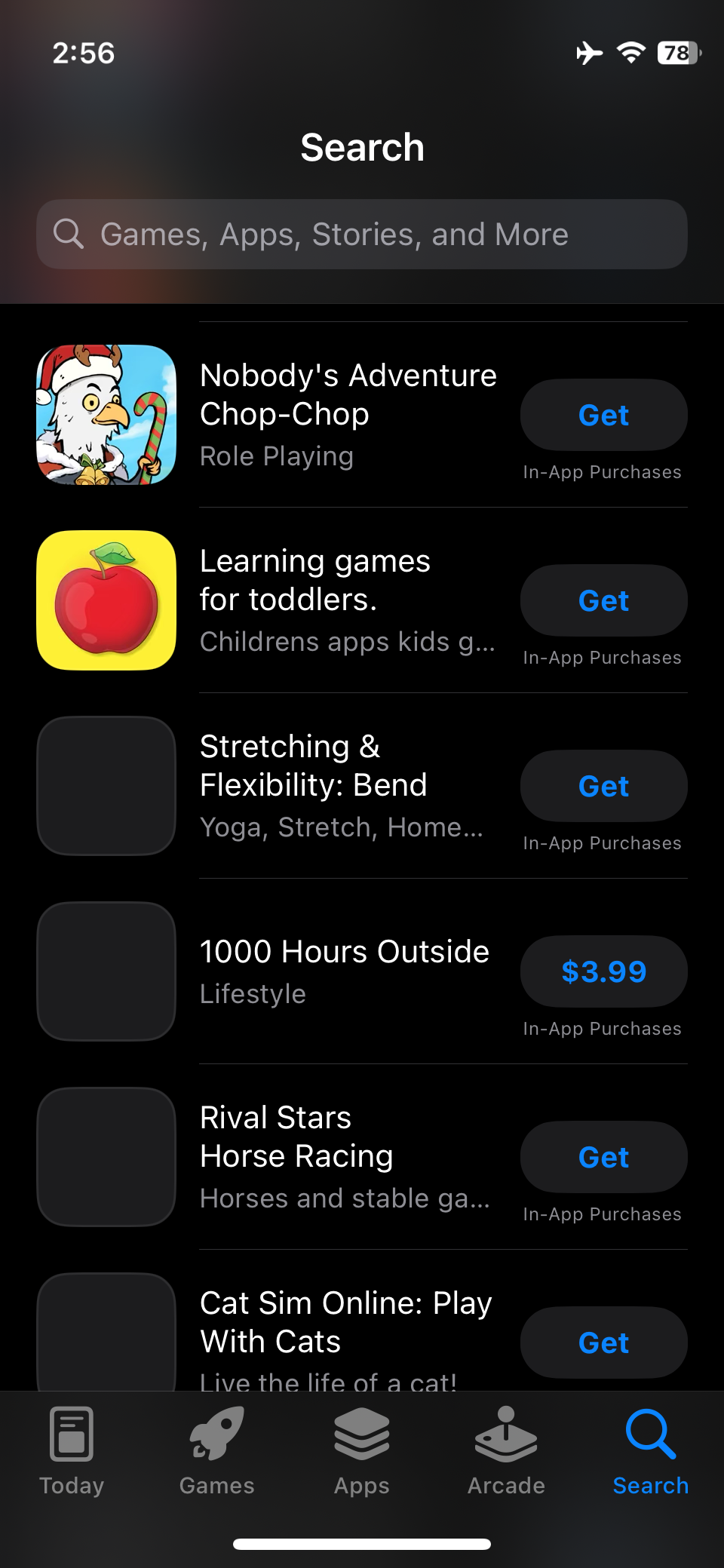A phone screenshot reveals various details on the device's interface. At the top left corner, the time is displayed as 2:56. On the right, the phone is in airplane mode, indicated by an airplane icon, followed by a fully lit Wi-Fi signal icon and a battery icon showing 78% charge, with '78' also displayed inside it.

In the center, the word "Search" is showcased, accompanied by a highlighted gray area with a magnifying glass icon. Below this search bar, tabs labeled "Games," "Apps," "Stories," and "More" are visible.

Underneath these tabs, there are placeholders for four images, of which two are filled. The first image is a cartoon drawing of an eagle holding a candy cane and wearing a Santa Claus hat, with the caption "Nobody's Adventure Chop-Chop" next to it, along with a "GET" button. The second filled image is a cartoon depiction of an apple, associated with the caption "Learning Games for Toddlers," also accompanied by a "GET" button.

Beneath these, listings show:
1. "Stretching and Flexibility" related to "1000 Hours Outside" with a price label of $3.99.
2. "Rival Stars Horse Racing."
3. "Cat Slim Online," encouraging users to "Play with Cats."

Lastly, at the very bottom of the screenshot, there are five icons arranged horizontally.